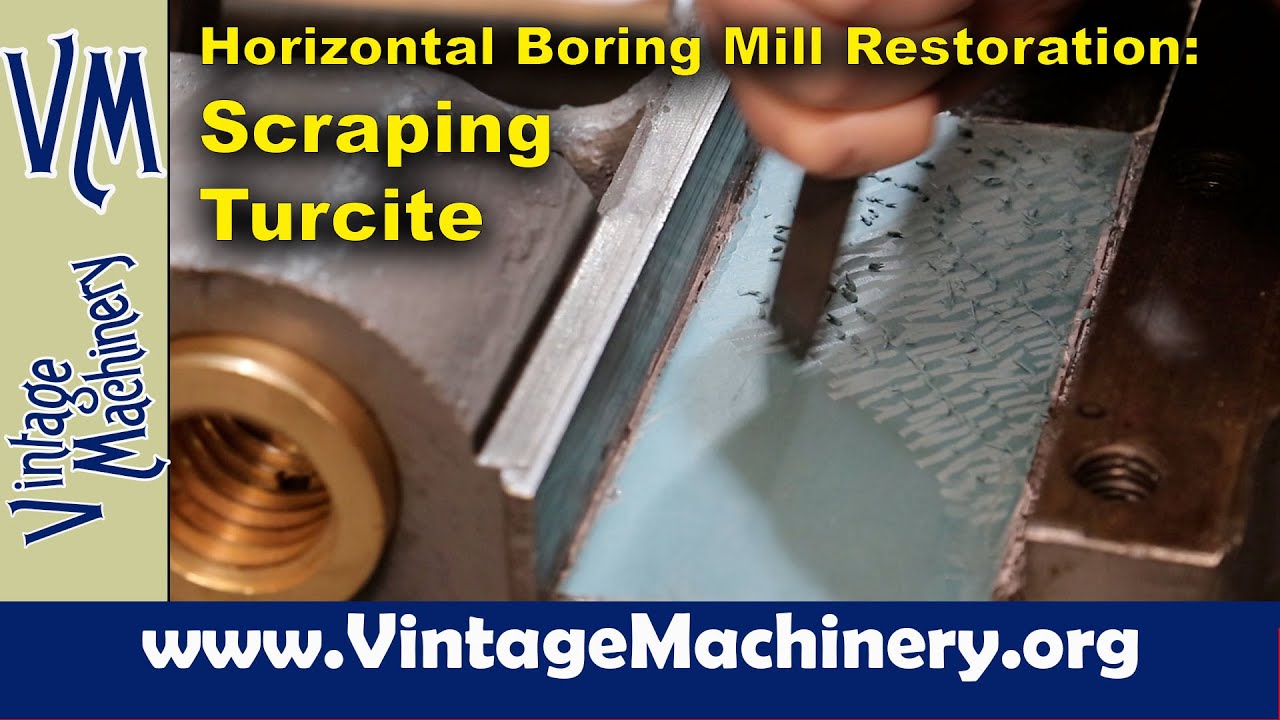This advertisement from Vintage Machinery prominently features a close-up image of a horizontal boring mill restoration process, specifically highlighting the technique of scraping Turcite. The top of the advertisement displays the header "Horizontal Boring Mill Restoration: Scraping Turcite" in yellow text. Beneath this, a photograph shows a partially visible, slightly blurry hand holding a chisel, seemingly engaged in scraping blue material from a greyish-blue metal surface. Along the left side of the ad, a vertical green banner with navy blue text and white outlines reads "VM" at the top and "Vintage Machinery" sideways below it. At the bottom of the advertisement, a blue horizontal bar contains the website URL, "www.vintagemachinery.org" in white text, linking back to the Vintage Machinery online platform. The overall design suggests a detailed, hands-on demonstration of vintage machinery restoration techniques.